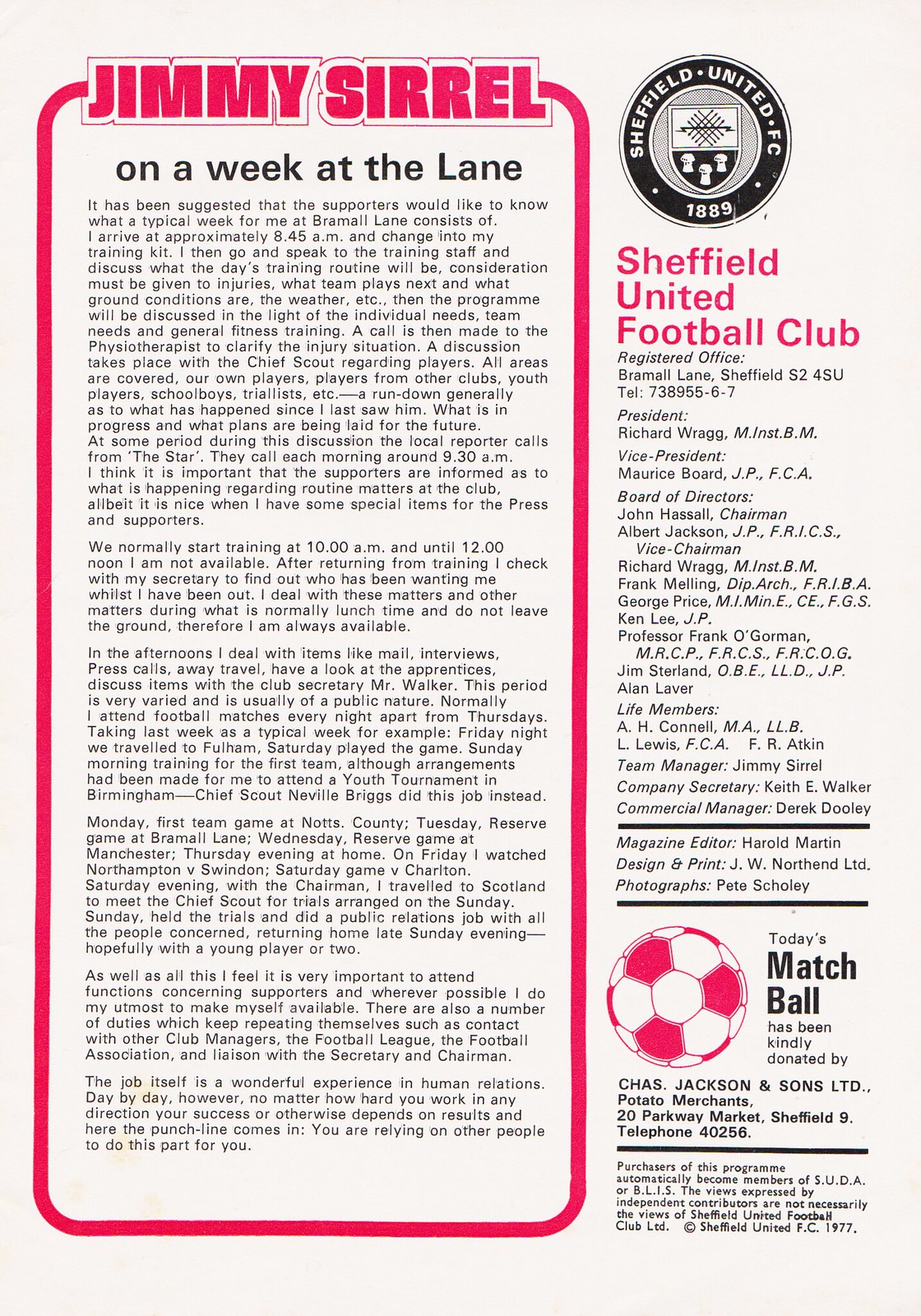The image is a detailed page from a magazine about Sheffield United Football Club, prominently featuring the title "Jimmy Searle" at the top. The page is rich with information about the club, displaying a circular logo bearing the text "Sheffield United FC, 1889." It details various administrative and managerial roles, including the President Richard Ragg, Vice President Maurice Board, and Team Manager Jimmy Searle, among others.

On the right side, under the heading "Registered Office," it lists the club's contact details and extensive information about the board of directors and key personnel. Featured prominently in the bottom right corner is an image of a red and white soccer ball with the caption stating it has been "kindly donated by Chaz Jackson & Sons Limited Potato Merchants."

The left side of the page showcases an article outlined in red titled "On a Week at the Lane." It provides an in-depth look at Jimmy Searle’s typical week at Bramble Lane, detailing his daily routine, interactions with staff, training schedules, and match preparations. The article delves into Searle's day-to-day activities, from morning training sessions to handling administrative duties, and his engagements with scouts, reporters, and supporters. It also recounts specific events from a recent week, highlighting the extensive travel and diverse responsibilities he manages, emphasizing his commitment to the club and its supporters. 

Overall, the page captures the organizational structure and daily operations of Sheffield United Football Club, providing a comprehensive insight into the life of Team Manager Jimmy Searle and the club’s activities.